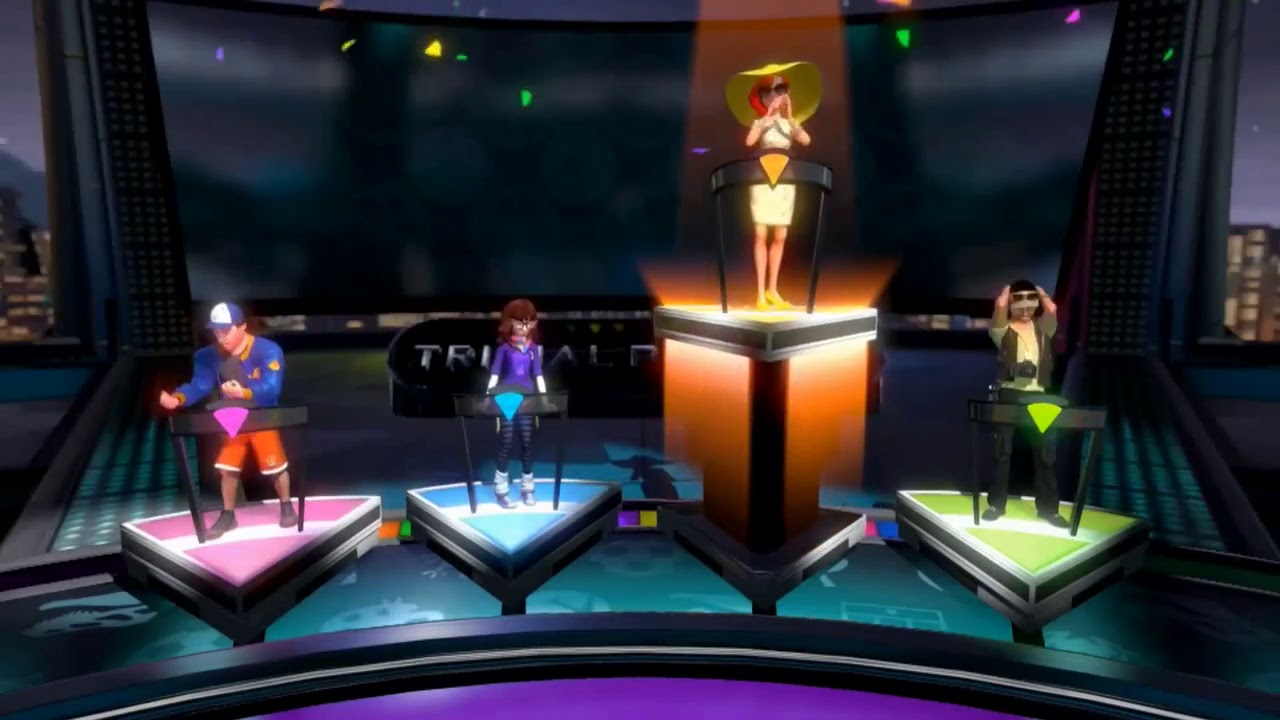This image is a vibrant screenshot from a video game that takes place in a virtual world. It depicts four characters positioned on triangular platforms, each navigating what seems to be a musical or DJ competition. The characters each stand in front of distinct podiums, possibly doubling as keyboards or control panels. The platforms are color coordinated: pink, blue, orange, and green, set on a larger stage with a dark backdrop.

The central figure, elevated above the others on an orange platform, is a woman with striking red hair, adorned in a yellow dress and a large yellow hat. To her right, a man stands on the green podium, recognizable by his black pants, black baseball cap, and sunglasses. On the far left, there is another male character donning orange shorts, a blue and white baseball cap, and a blue jacket. Adjacent to him, on the blue podium, is a young woman in a purple shirt with brown hair. All characters are distinctly styled, adding to the game's unique and dynamic atmosphere.